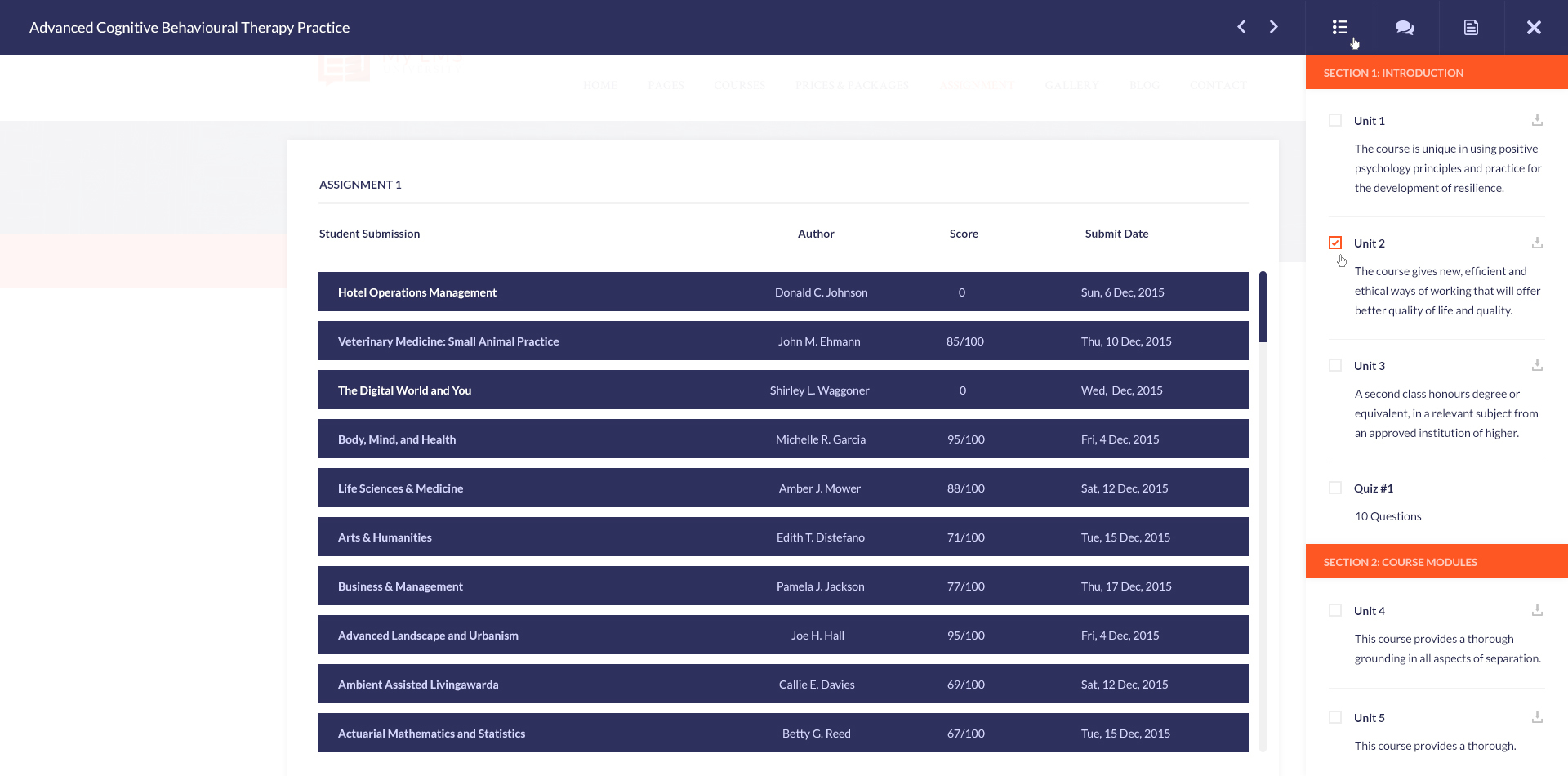The image displayed is a screenshot of a school's web page dedicated to an Advanced Cognitive Behavioral Therapy Practice course. The primary focus of the page is an educator's view of student assignments. At the center, a prominent rectangle labeled "Assignment 1" is visible, suggesting the specific task being reviewed. Below this, there are four distinct columns labeled "Student Submission," "Author Score," "Submit Date," and "Title." These columns contain data for approximately 10 to 11 student submissions, each row detailing individual entries with the student's submission title, the author's name, the score received, and the submission date.

On the far right of the page, there is a navigation bar titled "Session 1," with several entries listed beneath it: "Section 1 Introduction," "Unit 1," "Unit 2," "Unit 3," "Quiz 1," "Unit 4," and "Unit 5." The currently selected unit is "Unit 2," indicated by a highlighted or differently colored marker, implying that the presented assignments are related to this particular unit. This layout helps educators easily track where students are in the course and manage evaluations effectively.